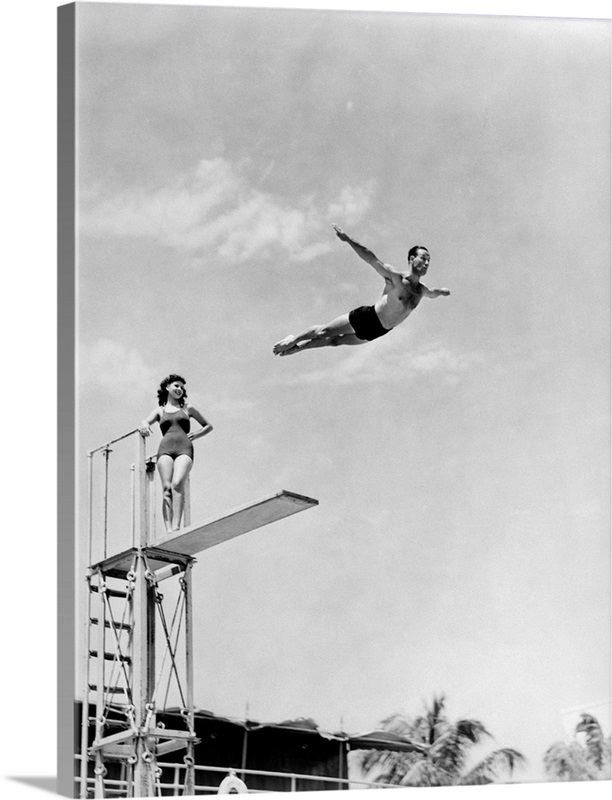A captivating vintage photograph captures a moment of grace and athleticism. In this black-and-white image, a Caucasian man is caught mid-dive from a high diving board. His form is impeccable; with arms extended outward like wings, toes pointed, and head held high, he epitomizes elegance and control. Below him on the springboard platform stands a woman, also attired in swimwear that suggests the 1950s. She wears an old-style bathing suit complemented by a period-appropriate hairstyle, further cementing the image's nostalgic aura. The overall scene exudes a timeless quality, transporting viewers back to a bygone era of simple pleasures and classic swimwear fashion.